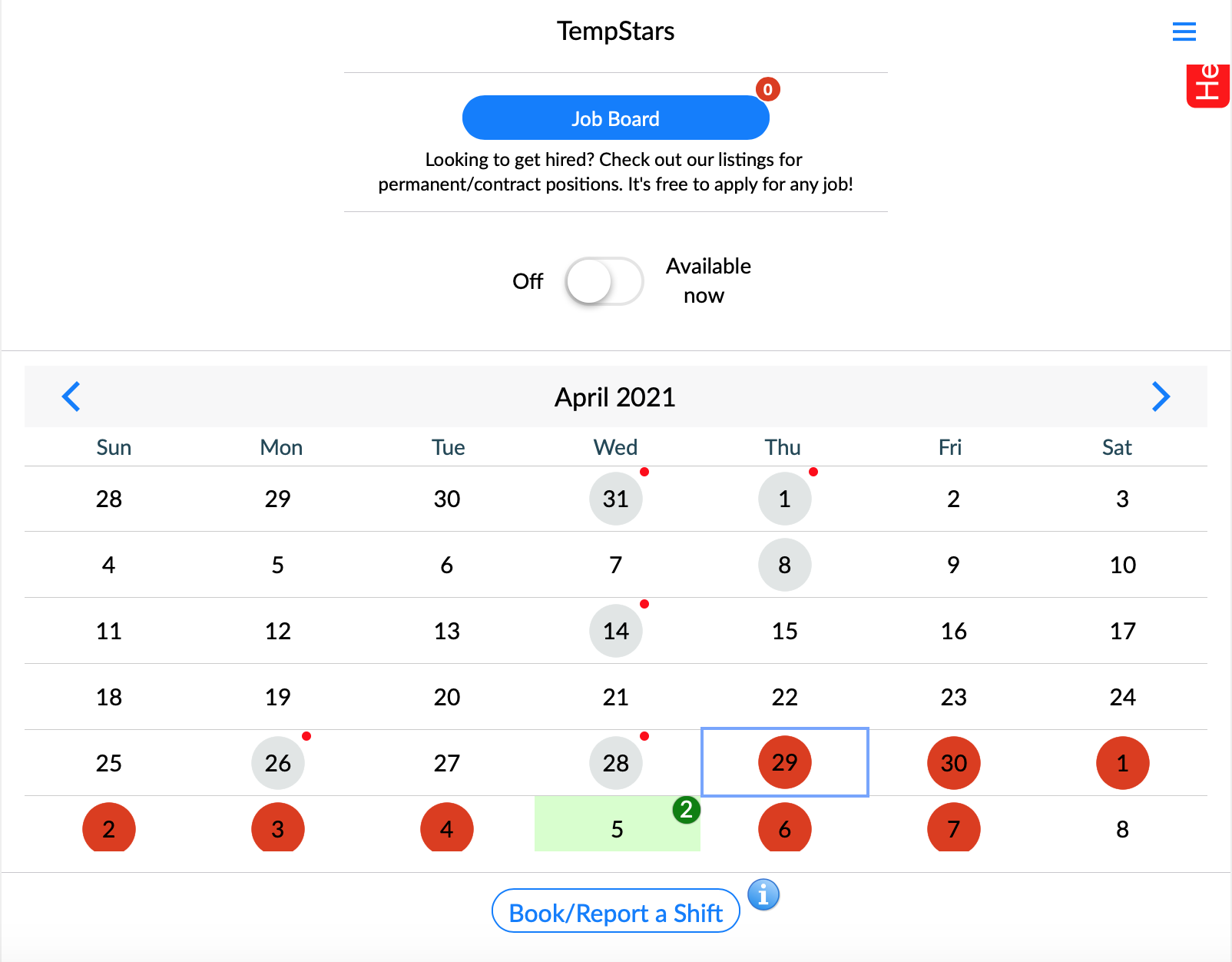This image depicts a computer screen displaying a job board interface from an application called "Temp Stars." The top section features a blue, rounded rectangle with the title "Job Board" printed in white text. Below this header, a prominent black text message reads: "Looking to get hired? Check out our listings for permanent contract positions. It's free to apply for any job."

Mid-screen, there is a slider control with a white ball currently set to the "off" position on the left side. The right side of the slider is labeled "Available Now," indicating the option to toggle availability status.

Towards the bottom of the screen, a calendar for April 2021 is visible. The days of the week are abbreviated as "Sun," "Mon," "Tue," "Wed," "Thu," "Fri," and "Sat." Various dates within the calendar have small dots in the corners, which are color-coded in red or gray. Additionally, the date "April 5th" is distinctly marked with a green rectangle surrounding it.